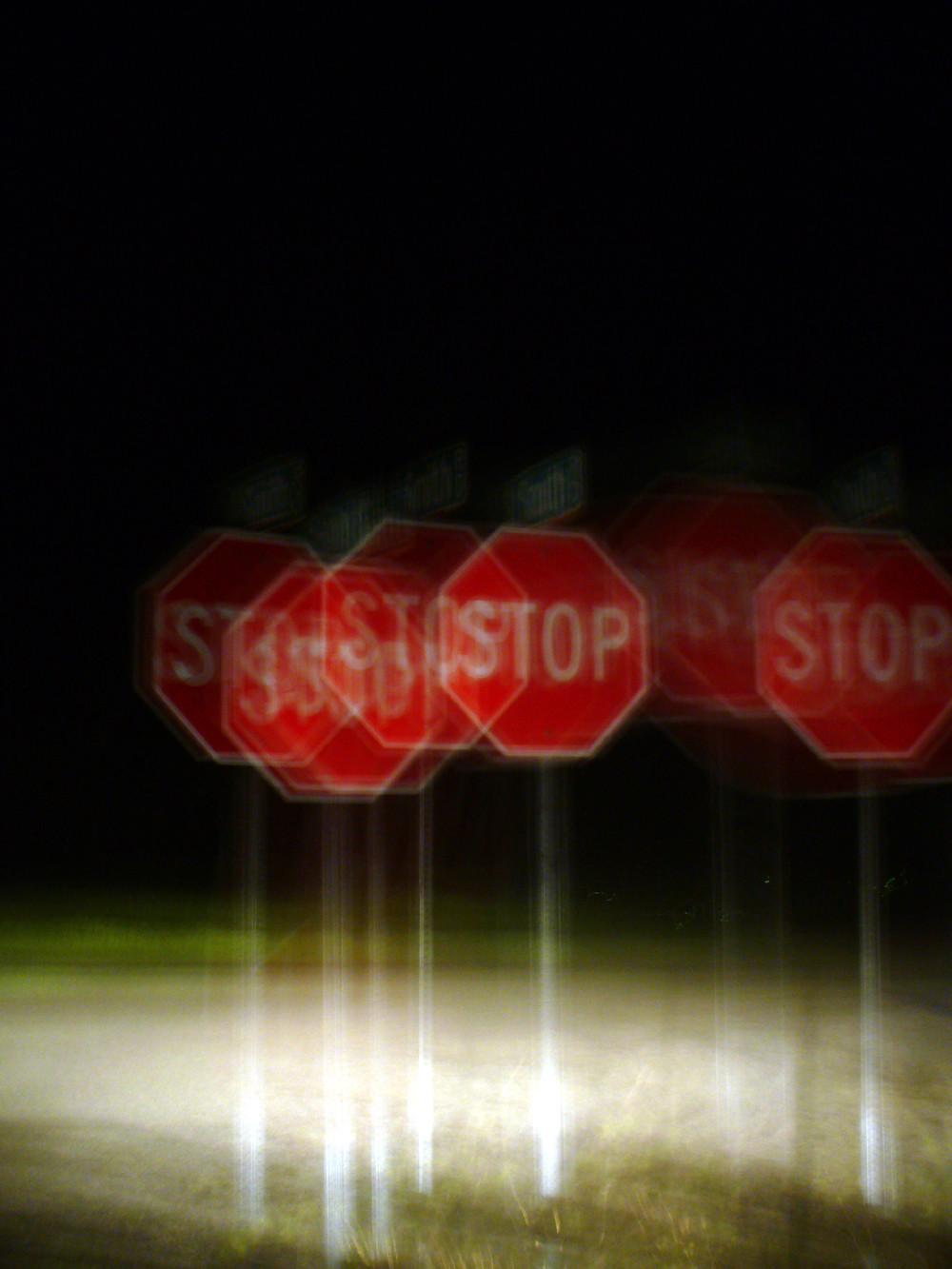The image, captured at night, features a blurry and somewhat surreal scene dominated by multiple superimposed images of what appears to be a single stop sign. The stop sign, mostly centered in the photo, shows a white and red color scheme with several ghostly replications surrounding it, creating the illusion of eight stop signs. To the right of the stop sign and slightly blurred is part of a street sign, which vaguely reads "South," though it's hard to discern clearly. The background is uniformly black with no visible stars, accentuating the effect of the bright, white headlights shining from the right, which illuminate the scene. Below the stop signs, there's a hint of green grass mixed with burnt brown patches. The poles of the stop signs reflect some of the ambient light, adding to the eerie and dreamlike quality of the photograph.